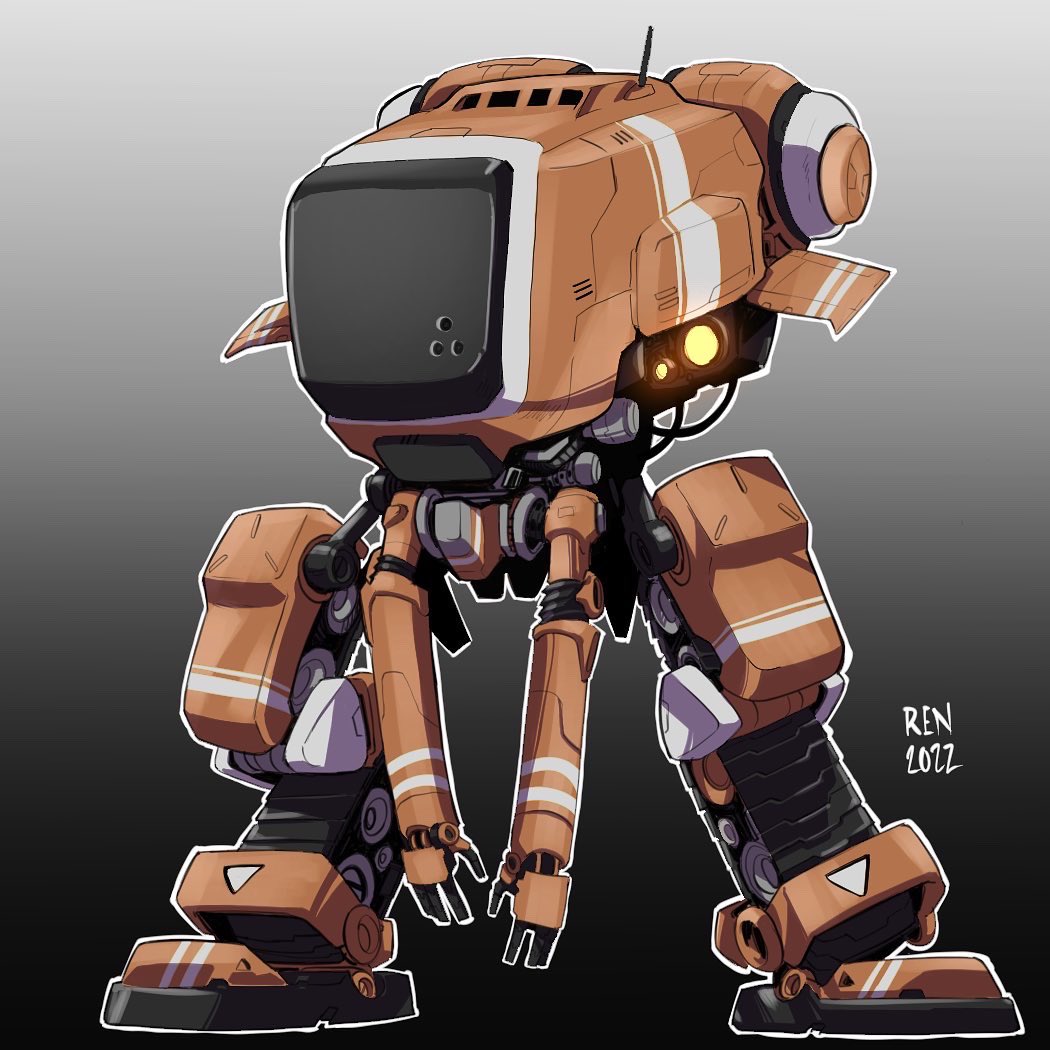This digital artwork features a futuristic, cartoon-style robot character with a unique and detailed design. The robot, primarily a muted brownish-beige color with white and black accents, has large, bulky legs and smaller arms that dangle down the front. The head and body resemble an old-fashioned, boxy TV screen with various cables and pieces extending from underneath. A yellow light is visible beneath the head, adding a touch of vibrancy. The robot has distinctive white stripes and triangles decorating its exterior. The image boasts a gradient background that transitions from dark gray at the bottom up to a lighter gray at the top, enhancing the focus on the central figure. Signed by the artist with "REN 2022" in a spidery white font on the right side, this piece suggests the robot could transform into different forms such as a car, airplane, or video camera.